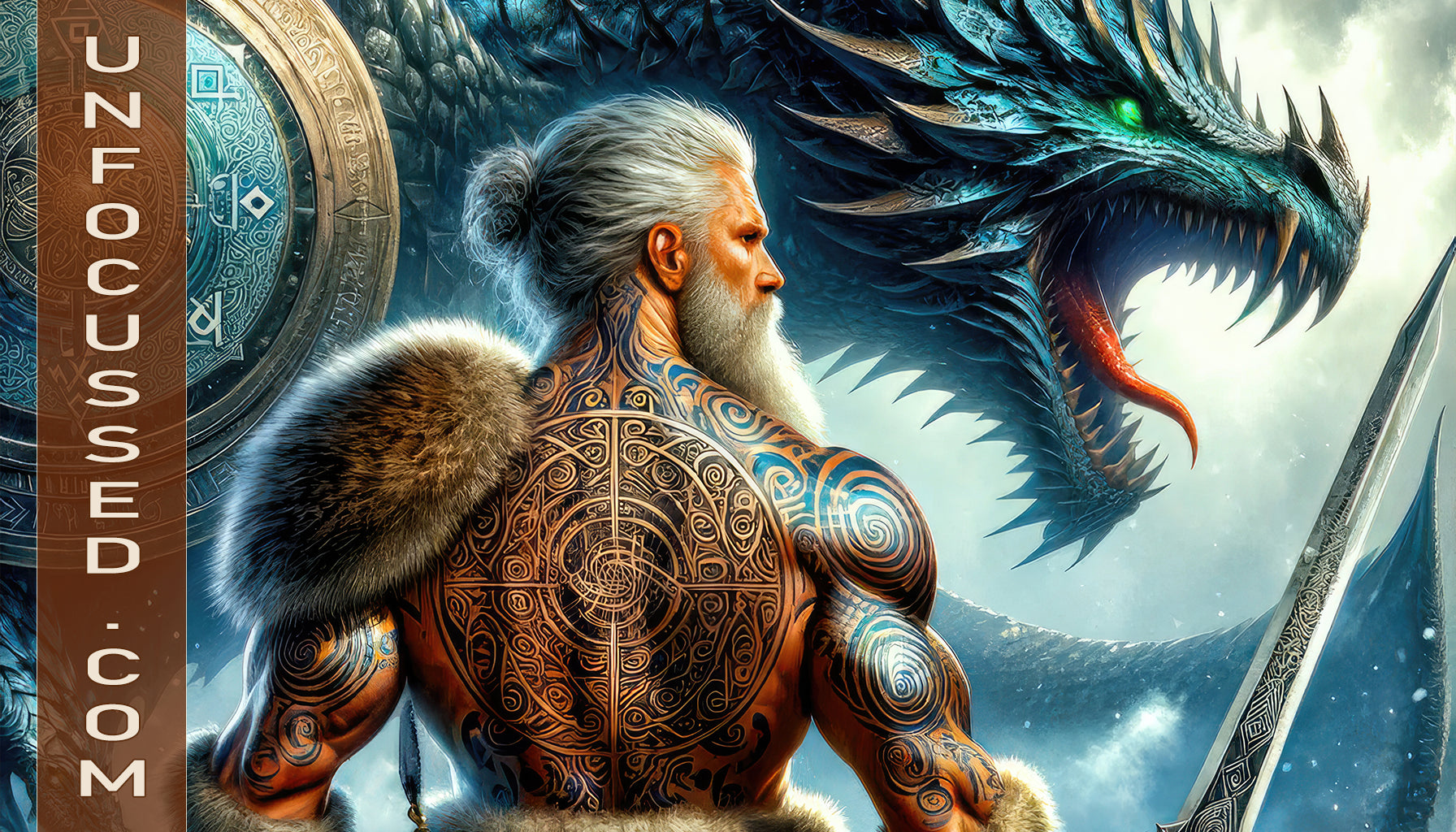The image is a rectangular, full-color illustration advertising the website "unfocussed.com" with vertical white text running from the top to the bottom on a brown banner along the left side. The drawing showcases a large, shirtless man viewed from the back. He has elaborate blue and black tattoos covering his arms and back. His long hair is tied back into a ponytail, and he sports a substantial gray beard. Draped over his left shoulder, he wears a piece of animal fur, matched by fur-trimmed gloves and a loincloth. In the bottom right corner, he firmly grasps a silver sword adorned with black decorations. The background prominently features a menacing dragon head with spikes, a red tongue, green eyes, and sharp teeth, rendered in hues of blue and purple, further enhancing the image's dramatic and fantastical aesthetic.